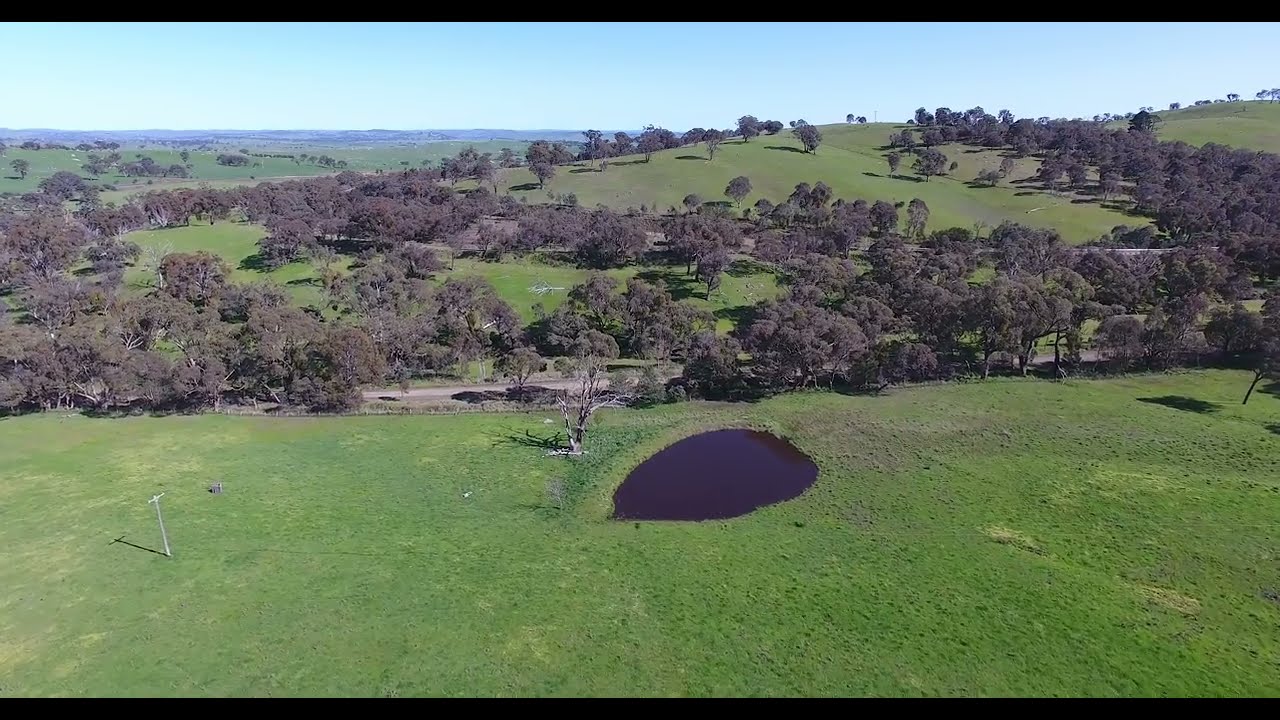The image captures a vast aerial landscape, likely taken from the height of a helicopter. It showcases a blend of nature's autumn hues with various trees flaunting yellow, brown, and purple leaves. Scattered dead trees, starkly white and brown, punctuate the occasional clearings filled with green and brown grass. These open fields weave through the trees haphazardly, hinting at an untamed, natural growth. In the distance, rolling hills mirror the diverse palette, with an asphalt road slicing through them horizontally about two-thirds up from the bottom of the image. Perched atop the far-right hill is a metal tower, standing sentinel over the scene. The top and bottom of the image are bordered by black bars, and the clear sunny day highlights the vivid contrast between the vibrant foliage and the serene sky.